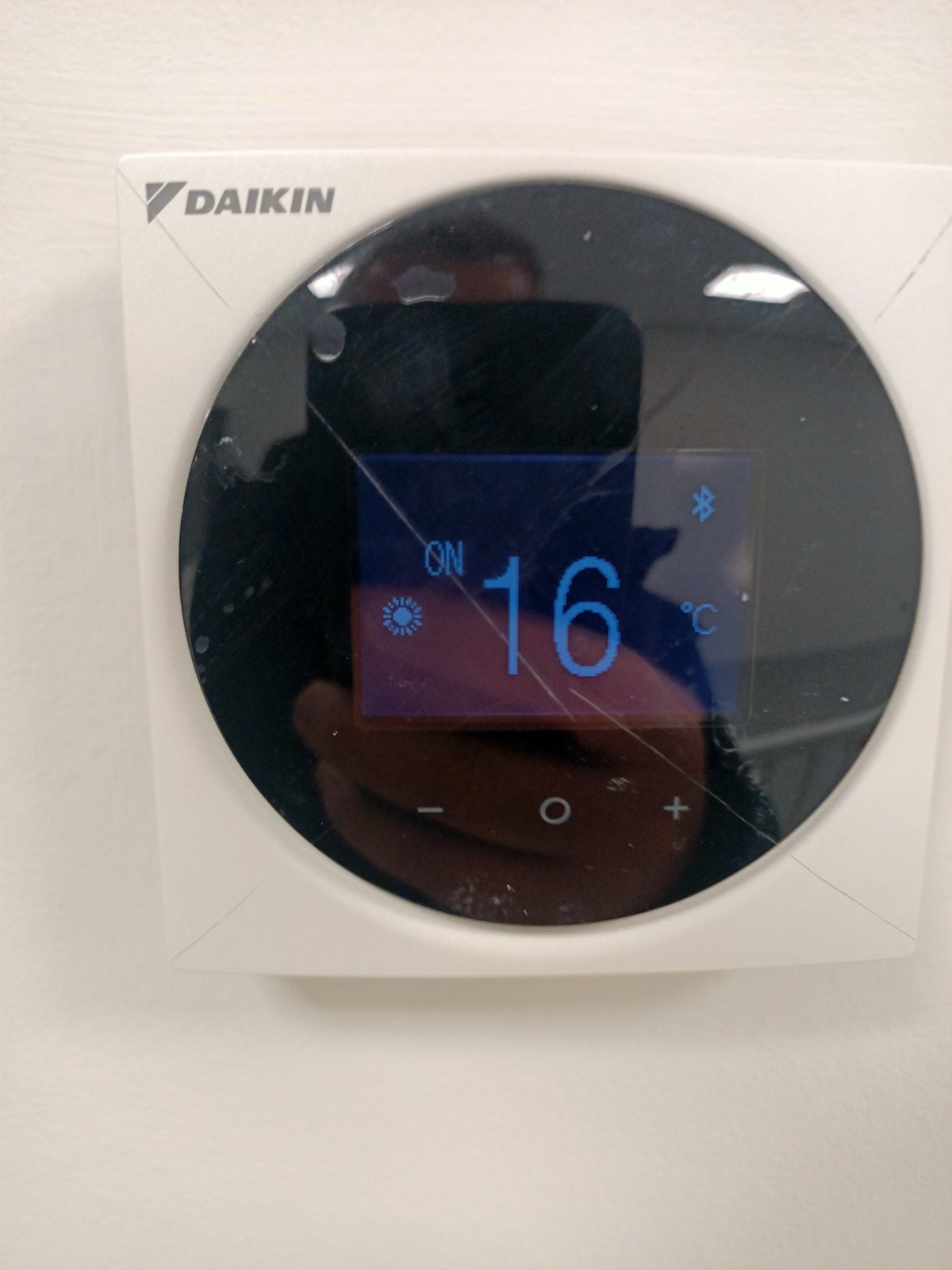This image showcases a Daikin smart thermostat situated in the top left-hand corner of the frame. The thermostat is encased in a white plastic square with a dome cover. The company logo, "DAIKIN," is prominently displayed in gray-black letters alongside a gray triangle. The device features a small LCD screen indicating a temperature of 16 degrees Celsius, with a Bluetooth symbol on the right side and a blue sunburst icon to the bottom left of the "on" status indicator. Below the screen are three tactile buttons: a minus sign, a circle, and a plus sign.

Notably, the thermostat is damaged, displaying a large crack that extends from the top left-hand corner to the bottom right-hand corner, along with several scratches and scuffs. Reflecting on the dome cover, the image captures the person taking the photograph—a man with brown hair and a slightly receding hairline, holding a camera up to his face. The setting appears to be an office, and the entire scene is framed against a white background.